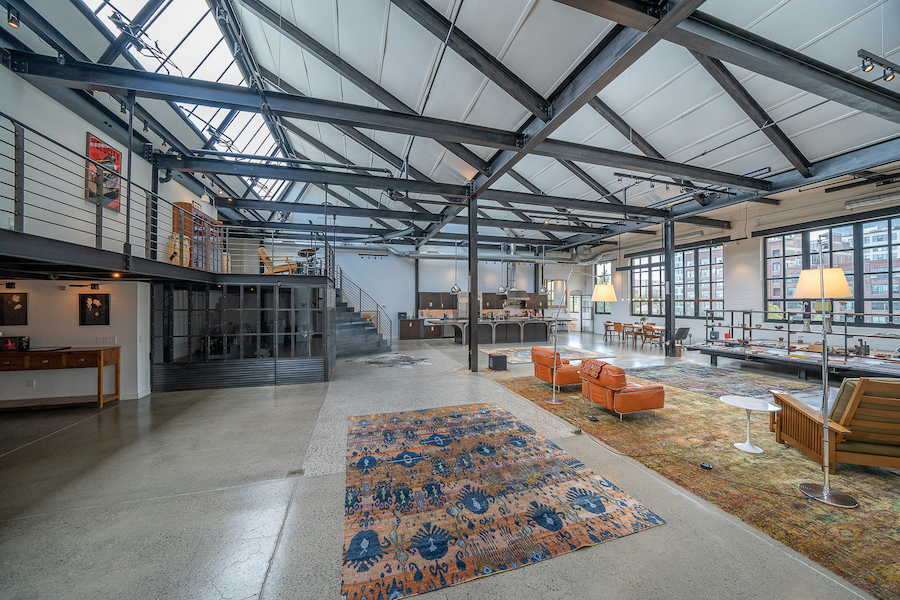This photograph showcases a spacious, open concept loft with a mix of modern industrial design elements and cozy, curated furnishings. The large room is segmented into distinct areas, each defined by vibrant area rugs and functional decor. Central to the room is a dark blue and orange patterned rug with seating arrangements comprising orange love seats and green chairs around white tables, all illuminated by tall, silver floor lamps. Nearby is a wooden lounge chair next to an oval-topped end table.

On the left side of the room, a wooden console table or desk is lined against the wall, adorned with photos of people in black clothes above it. The room also features a lofted second level accessible via a long, steel staircase, adding to the industrial ambiance with visible steel beams and columns. The upstairs area contains a chair and bookcases, providing a cozy reading nook that overlooks the main living space.

At the far back of the room is a fully-equipped kitchen with dark brown cabinetry, a peach-colored backsplash, a stainless steel hood, and a kitchen island with bar seating. High-top tables occupy the space near the kitchen, enhancing the open layout. The expansive windows along the right wall flood the area with natural light and offer views of neighboring brick buildings and trees, contributing to the bright and airy feel of the environment. The mix of industrial elements with warm, personal touches makes this loft both stylish and inviting.